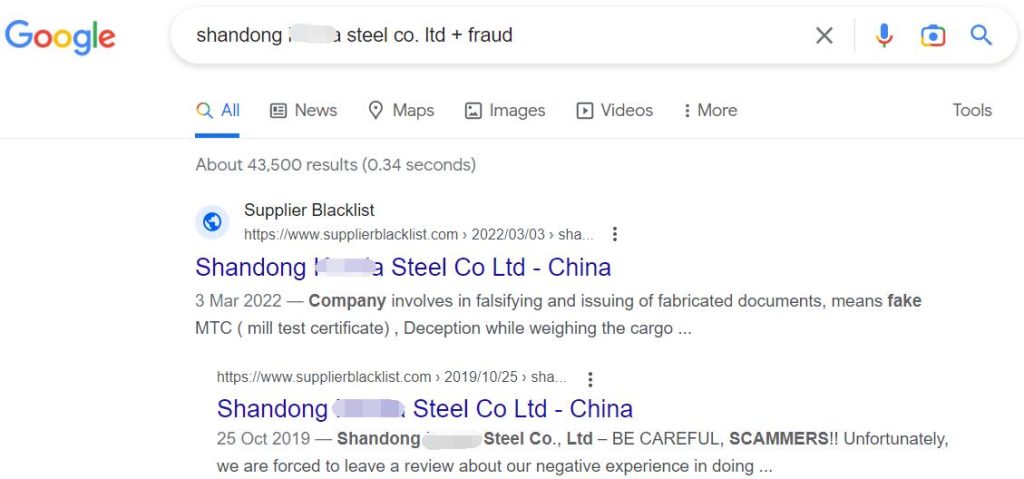The image is a detailed screenshot of a Google search results page. In the top left corner, the recognizable Google icon is prominently displayed. Next to the icon, spanning most of the width of the page, is the search bar. The search query entered is "Shandong [blurred word] Steal, Co, Limited + Fraud," with the second word in the phrase manually rubbed out in gray, rendering it unreadable.

Below the search bar are several navigation tabs including "All," "News," "Maps," "Images," "Videos," "More," and "Tools," all accompanied by their respective icons. The "All" tab is highlighted in blue, indicating it is the active tab.

Immediately beneath these tabs, the search results begin. The first result reads "About 43,500 results (0.34 seconds)," indicating the number of search results and the time taken to generate them. The top result is marked with a globe icon inside a circle, labeled "Supplier Blacklist." 

The listing's website address follows alongside the partly obscured company name: "Shandong [blurred word] Steal, Co, Limited, China." The entry is dated 3 March 2022 and includes text stating: "Company involved in falsifying and issuing fabricated documents, including fake MTC (Mill Test Certificate) and deception while weighing the cargo."

Included within this main listing is a subcategory, with a slightly indented text that also includes the company name "Shandong [blurred word] Steal, Co, Limited, China," but this time dated 25 October 2019. The following review warns: "Be careful, scammers. Unfortunately we are forced to leave a review about our negative experience in doing..."

The image captures a detailed account of a potentially fraudulent company with emphasis on negative reviews and warnings about deceptive business practices.